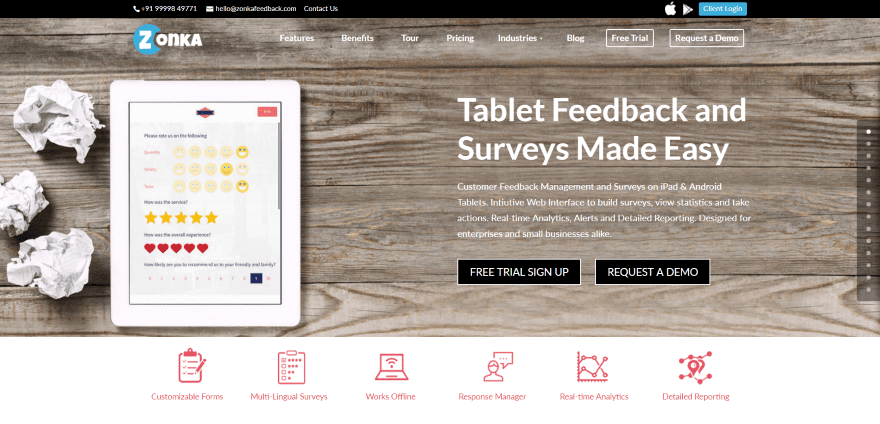**Website Screenshot Description:**

The screenshot captures a webpage from the Zonka website. The topmost bar is thin and black, featuring a small phone number, a website link, and the "Contact Us" option, all in diminutive print. Additionally, the bar includes the Apple icon, a right arrow, and a "Client Login" box.

The central focal point of the webpage is a professionally designed logo: a blue circle with a white "Z" followed by "O-N-K-A" in text. Below the logo, the primary navigation menu offers various selections including: Features, Benefits, Tour, Pricing, Industries, Blog, Free Trial, and Request a Demo.

The main section of the image showcases a white iPad placed on a rustic wooden desk, accompanied by several crumpled pieces of paper scattered around. Prominently displayed on the iPad screen, in bold white print, is the slogan: "Tablet feedback and surveys made easy."

Smaller text adjacent to the iPad provides further context: "Customer feedback management and surveys on iPad and Android tablets. Intuitive web interface to build surveys, view statistics, and take actions. Real-time analytics, alerts, and detailed reporting designed for enterprises and small businesses alike." The page emphasizes the options to sign up for a free trial or request a demo.

At the bottom of the screen, additional features are highlighted, including: Customizable Forms, Multilingual Surveys, Works Offline, Response Manager, Real-time Analytics, and Detailed Reporting.